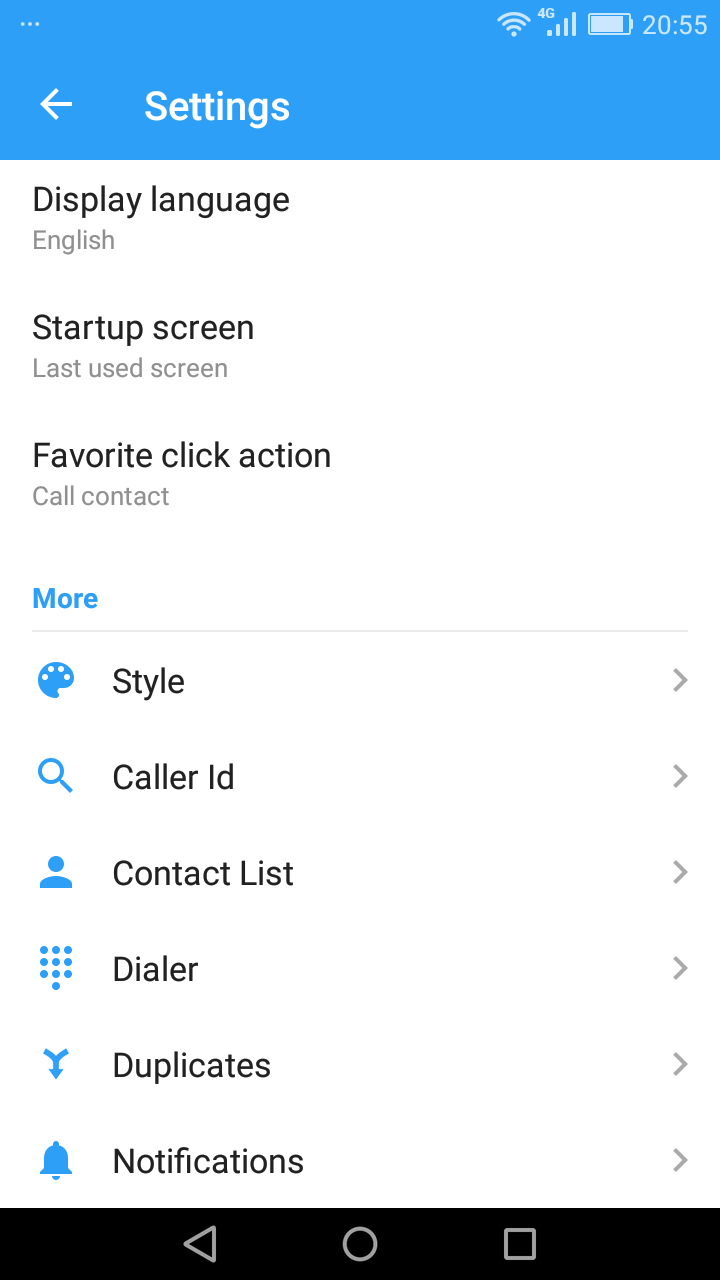Screenshot of a mobile phone settings page captured at 20:55. At the top, the status bar indicates that Wi-Fi is enabled and the battery level is nearly full. The central part of the screen features a heading "Settings" in a blue bar. Below the heading, the screen displays several options: 

- **Display Language**: Set to English.
- **Startup Screen**: Configured to the "Last Used Screen".
- **Favorite Click Action**: Assigned to "Call Contact".

Below these options, several expandable sections are shown, each with a blue icon and an arrow indicating further selections:

- **More Style**: Represented by a blue paint palette icon.
- **Caller ID**: Indicated with a magnifying glass icon.
- **Contact List**: Featuring an icon of a blue head and shoulders silhouette of a person.
- **Dialer**: Shown with a blue phone dial pad icon.
- **Duplicates**: Illustrated by two converging lines forming an arrow pointing down.
- **Notifications**: Represented with a blue bell icon.

Finally, a black navigation bar is present at the bottom, offering quick access to go back or return to the home screen, exhibiting a minimalistic design.